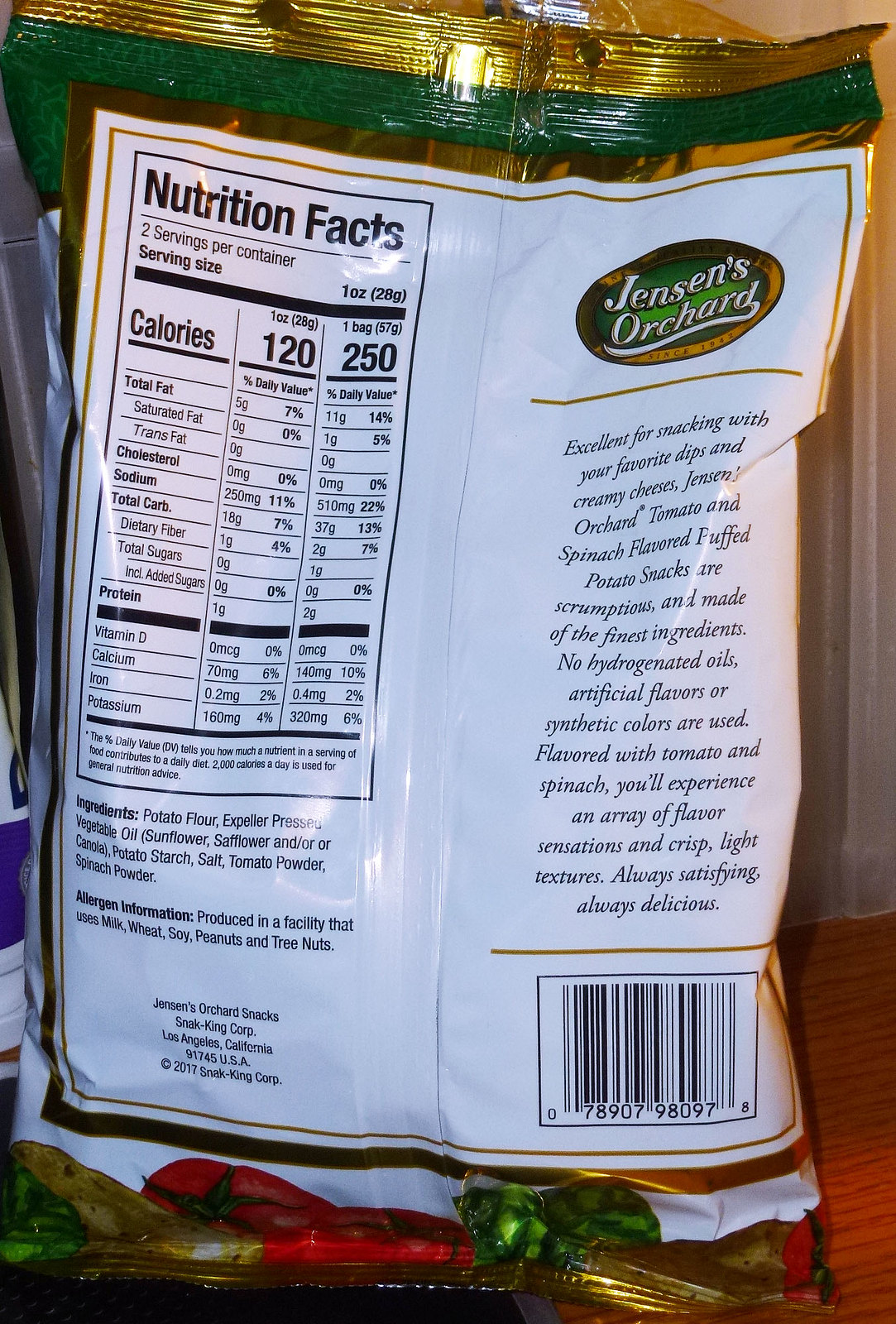In the image, we see the back side of a product package, clearly branded with "Jensen's Orchard" at the top. The packaging prominently features the word "Excellence." In the upper left-hand section, the Nutrition Facts panel indicates there are two servings per container, with each serving containing 120 calories, totaling 240 calories for the entire bag. The rest of the nutritional information is blurred and difficult to read. The majority of the package is white, with a barcode situated in the lower right-hand corner. Among the ingredients listed, potato flour appears to be the main component, suggesting the product might be potato chips.